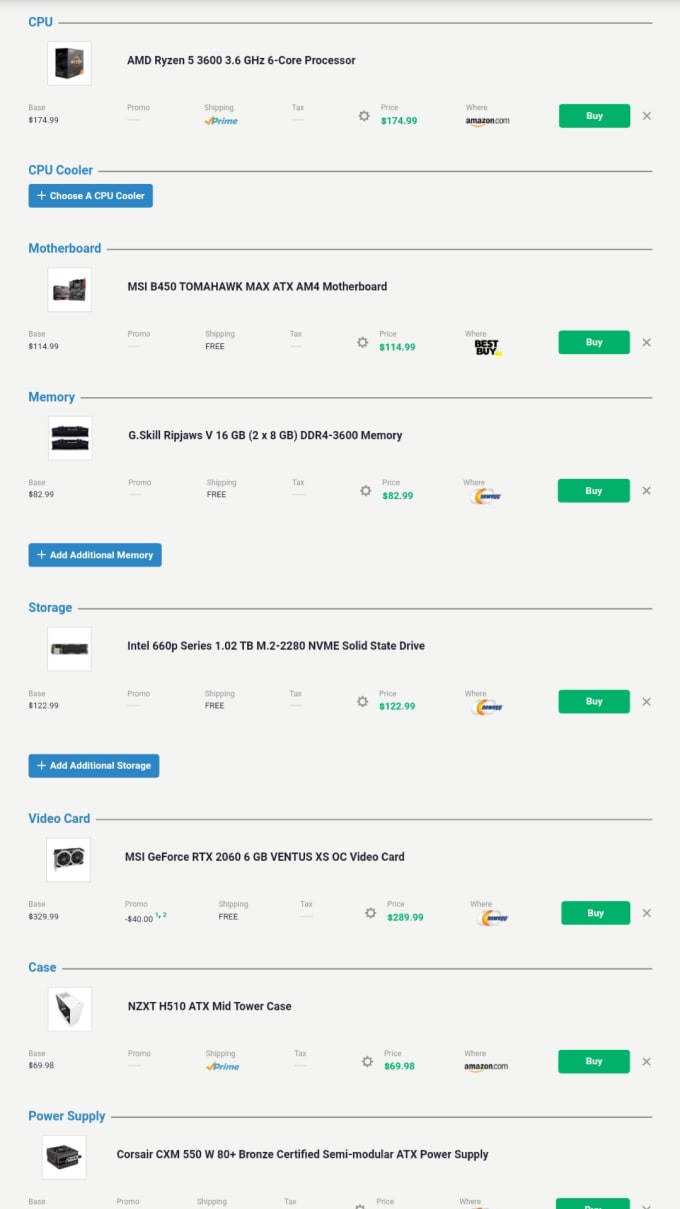This screenshot depicts a well-organized PC build list on a website similar to PCPartPicker, used for assembling a custom computer. Each component's selection is itemized with detailed pricing, shipping options, and purchasing sources:

1. **CPU**: The chosen processor is an AMD Ryzen 5 3600, a 6-core CPU priced at $174.99. It is available on Amazon with Prime shipping, accessible via a green "Buy" button.
   
2. **CPU Cooler**: No CPU cooler is selected. A notable blue "Choose a CPU Cooler" button prompts the user to add this item.

3. **Motherboard**: The build includes an MSI B450 Tomahawk Max ATX AM4 motherboard, costing $114.99. This item ships for free from Best Buy.

4. **Memory**: Selected memory consists of G.Skill Ripjaws V series 16GB DDR4, priced at $82.99, with free shipping from Newegg. There's also an option to add more memory through a corresponding button.

5. **Storage**: An Intel 660P Series SSD is chosen for storage, priced at $122.99. It also comes with free shipping from Newegg.

6. **Video Card**: The graphics card listed is an MSI GeForce RTX 2060. Initially priced at $329.99, it includes a $40 promotional discount, reducing the final price to $289.99, with free shipping from Newegg.

7. **Case**: The computer case is a NZXT H510 ATX mid-tower, priced at $69.98 and available from Amazon with Prime shipping.

8. **Power Supply**: The selected power supply is a Corsair CXM 550W 80 PLUS Bronze certified semi-modular ATX unit. However, the price is not visible in the screenshot.

This detailed list ensures a beginner or experienced builder can source each component efficiently, considering cost and shipping preferences.